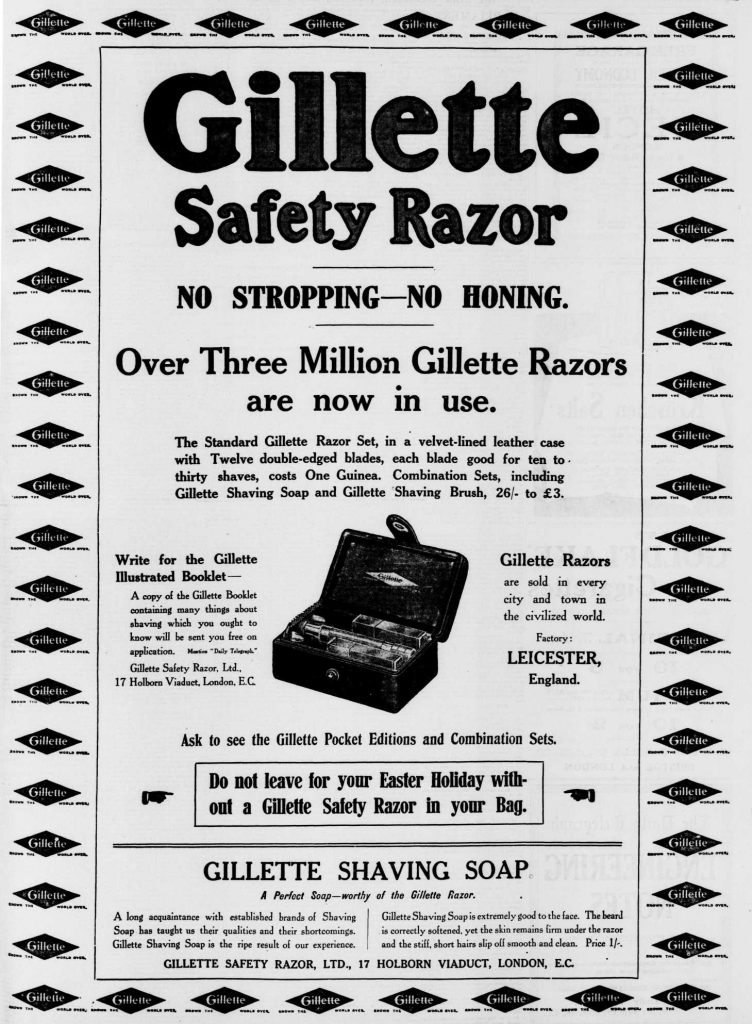This vintage advertisement for Gillette safety razors is presented in a black-and-white format. The ad is framed with a rectangular border adorned with the Gillette logo in a continuous pattern. Prominently displayed at the top in large, bold letters are the words, "Gillette Safety Razor - No Stropping, No Honing." It proudly states, "Over 3 million Gillette razors are now in use." The main focus is on the standard Gillette razor set, which includes a velvet-lined leather case and twelve double-edged blades, with each blade providing 10 to 30 shaves. The ad specifies that the set costs one guinea, and mentions combination sets that include Gillette shaving soap and a Gillette shaving brush, priced between 26 shillings to 3 pounds. A small image within the advertisement showcases an open razor case displaying the razors. Notably, the text reads, "Do not leave for your Easter holiday without a Gillette safety razor in your bag." Additional text in smaller print mentions features of the Gillette pocket editions and combination sets, as well as a description of the Gillette shaving soap as a perfect complement to the razor. Although some text is faint and difficult to read, the ad is rich with details emphasizing the convenience and popularity of Gillette products.